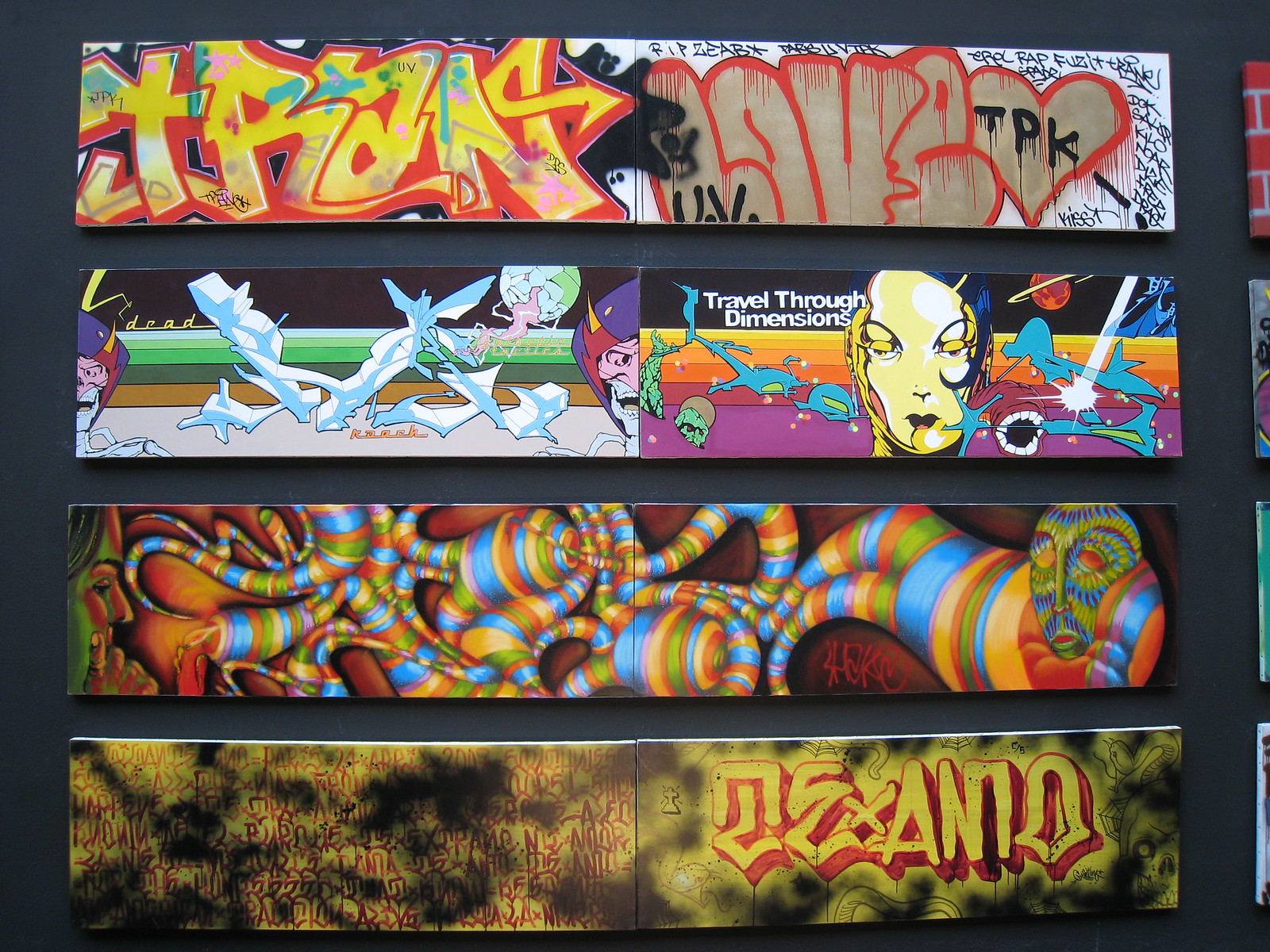This image showcases a series of graffiti art panels arranged horizontally against a black background, forming a striking visual narrative across four separate canvases. The topmost panel features vibrant yellow graffiti letters, possibly spelling "Trans Love," juxtaposed with brownish-yellow text set in a large, dynamic font. This graffiti is complemented by black-and-white script and accompanied by a heart motif on the right. Below this text-rich panel is an enigmatic structural illustration, visually complex and less graffiti-like.

The second panel presents a fantastical scene featuring a golden-hued female cyborg with black hair, flanked by monstrous figures. The phrase "Travel Through Dimensions" is inscribed to the left of her head, set against a backdrop that suggests interdimensional travel and otherworldly elements. This panel blends fantasy with sci-fi elements, incorporating planets and cosmic imagery.

Moving to the third panel, a surreal, tubular creature with a rainbow-colored, segmented body dominates the space. A figure holding a flame appears to be interacting with this trippy, extensive worm-like entity, which tapers off into a faceless, green-and-blue masked visage on the far right, evoking an eerie yet colorful effect.

The bottom panel returns to traditional graffiti motifs, marked by a grungy aesthetic. On the left side, the artwork is obfuscated by dark shadows, with symbols partially visible against a blotchy black background. The right side features the word "Texano" in bold yellow graffiti-style print outlined in red, encapsulating the gritty essence of street art.

Overall, these panels collectively weave a rich tapestry of graffiti art, fantasy illustrations, and surreal imagery, each contributing to a vivid and multifaceted visual experience.